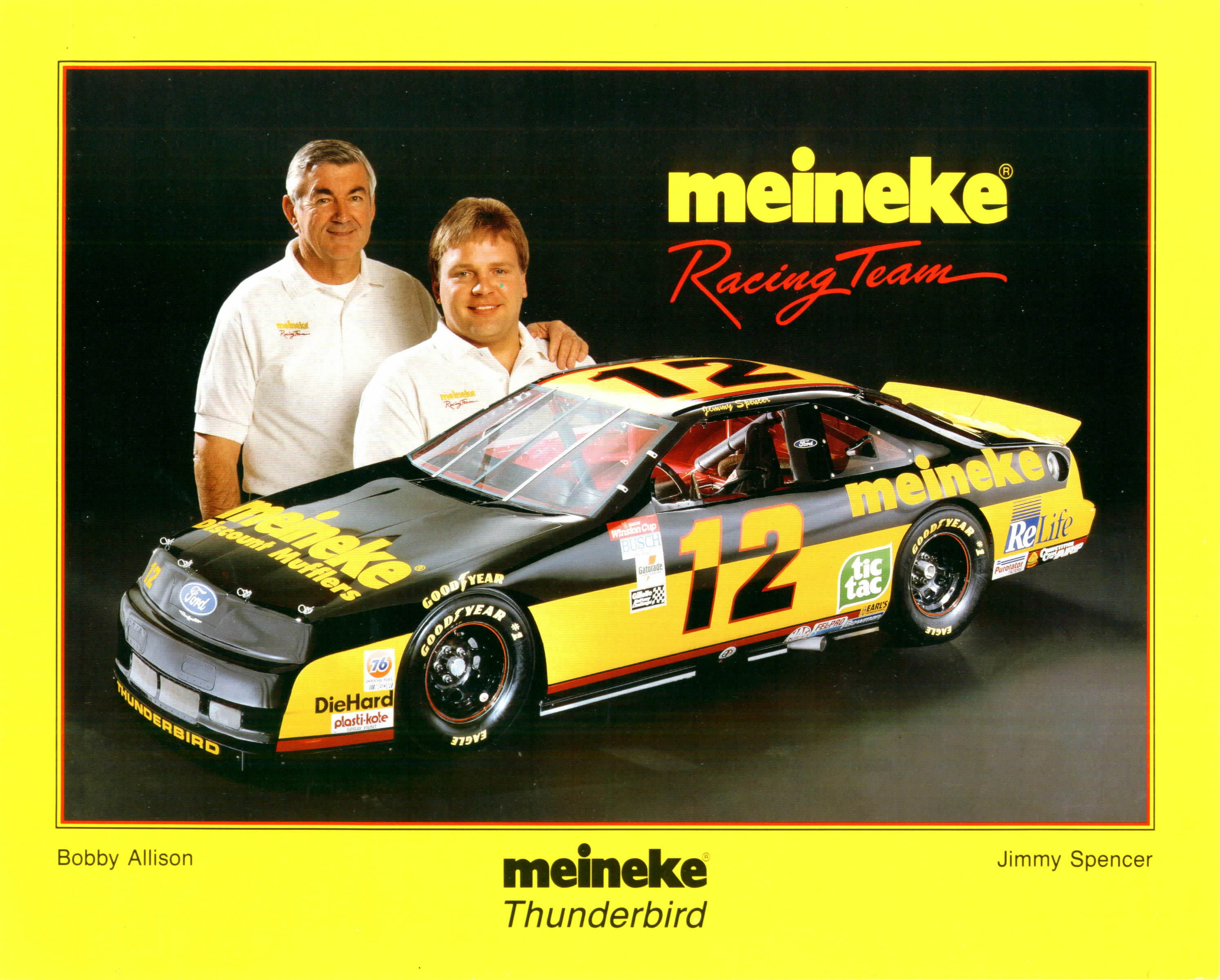This is a horizontally aligned rectangular poster with a yellow border that is especially thicker at the bottom. The lower left-hand corner features "Bobby Allison" in black text and the lower right-hand corner shows "Jimmy Spencer" in black text. Centered underneath the image, it says "Meineke" in bold black letters with "Thunderbird" below it. The poster displays a large photograph of a black and yellow race car with the number 12 prominently shown on the roof and side. The car has "Meineke Discount Mufflers" written in yellow on the hood, and various sponsor logos, including Tic Tac and Relife, positioned around the car. 

The upper right-hand corner of the poster has "Meineke" in bubble yellow letters and "Racing Team" in red cursive beneath it. Against a solid black background, the upper left-hand part of the image features two men. The older man, a white male with short salt-and-pepper hair, is smiling and has his left arm around the younger man, who has short brown hair and is also smiling with his teeth showing. Both men are wearing white Meineke polo shirts, with the older man's shirt displaying the Meineke logo on the right chest area. The car's front grill also shows the Ford emblem in blue and white. The photograph of the men appears to have been digitally added as they are notably larger than the car in the image, shown from approximately the torso up.